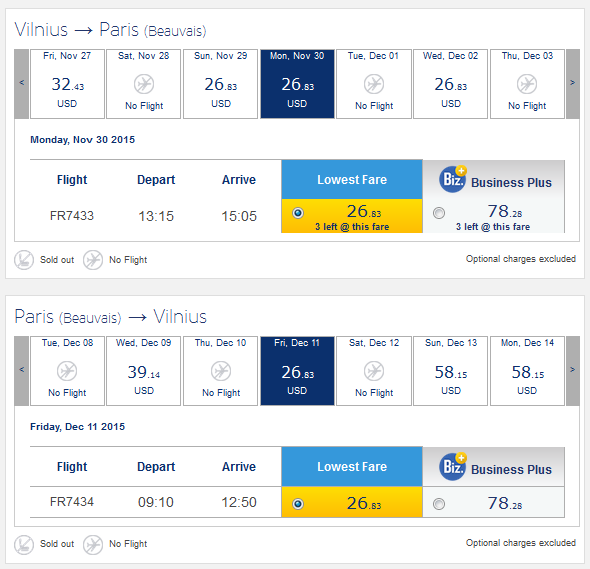The image displays detailed flight information for two separate routes between Vilnius (VILNIUS) and Paris (Beauvais). Here's a structured summary of the flight details:

**Vilnius to Paris (Beauvais):**

- **Travel Dates:** Friday, November 27th to Thursday, December 3rd, 2015.
- **No Flights:** Saturday, Tuesday, and Thursday.
- **Selected Flight:** Monday, November 30th, highlighted in a dark blue square showing a fare of $26.53 USD.
- **Flight Information for Selected Date:**
  - Date: Monday, November 30th, 2015
  - Depart and Arrive times available
  - Lowest fare is $26.53 USD
  - Price and amenities for Business Plus also displayed.
- **Visual Elements:**
  - Top section in blue indicates standard fare
  - Bottom section in yellow suggests Business Plus details.

**Paris (Beauvais) to Vilnius:**

- **Travel Dates:** Tuesday, December 8th to Monday, December 14th, 2015.
- **No Flights:** Tuesday, Thursday, and Saturday.
- **Selected Flight:** Friday, December 11th, highlighted in a dark blue square.
- **Flight Information for Selected Date:**
  - Date: Friday, December 11th, 2015
  - Depart and Arrive times available
  - Lowest fare displayed
  - Price and amenities for Business Plus also shown.
- **Visual Elements:**
  - Fair structure similar to the previous route, with visual highlights indicating relevant sections.

**Additional Information:**

- Optional charges are excluded from the displayed prices.

This detailed breakdown emphasizes the selected flights, their fares, and availability for each day within the described date ranges.